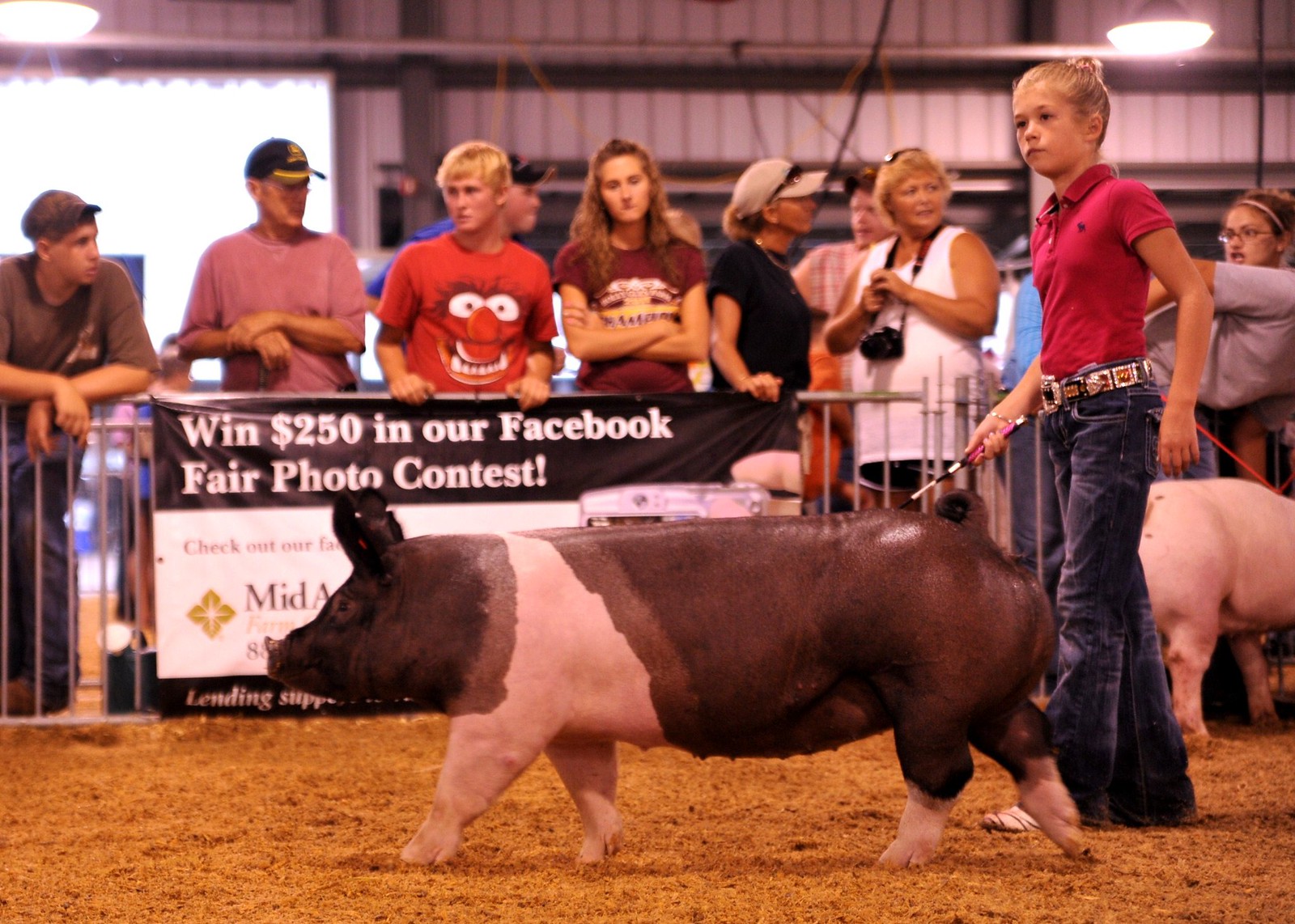The photograph captures a vibrant scene at a county fair, set within a convention space featuring a dirt floor and bustling activity. At the forefront stands a young girl, around 8 to 12 years old, with blonde hair neatly tied up in a bun. She wears a red polo shirt, dark bell-bottom jeans, and a large buckled silver belt. In her left hand, she holds a prod, which she uses to guide a large black and white pig to her left. The pig, with a mostly black body, white legs, and distinctive white markings behind its head, dominates the center of the image.

Immediately behind the young girl and to the right of the frame, the back half of another all-pink pig is barely visible. The background is lined with a fence adorned with a banner that announces, "Win $250 in our Facebook Fair Photo Contest." Spectators behind the barrier, most appearing to be college-age, include a variety of individuals engaged in conversation or watching the competition. Notable figures in the crowd are a man in a brown shirt with a ball cap, a young man wearing a shirt with a monster face, a bored-looking young lady with arms crossed, and a duo of women chatting, one in a black shirt and cap and the other in a white shirt with a camera around her neck. The overall atmosphere is lively and competitive, characteristic of a traditional county fair.